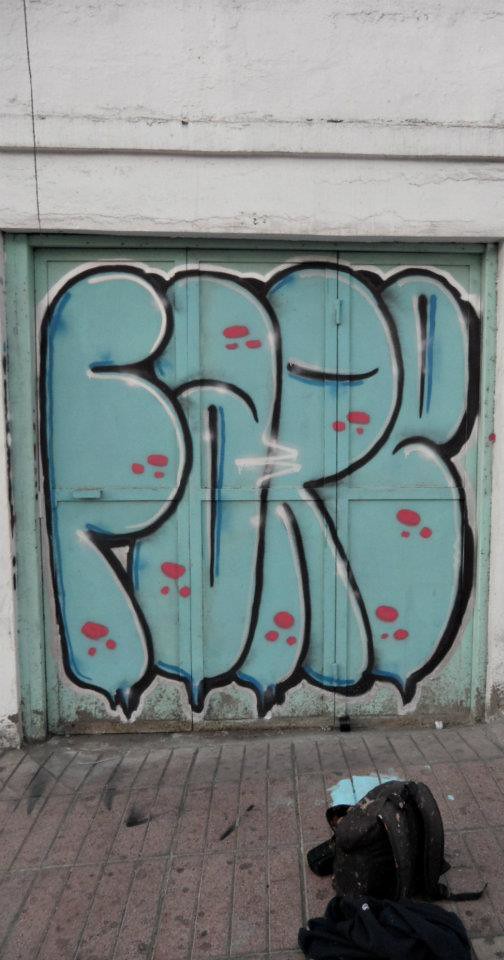The photograph captures a piece of graffiti art in the center of a decrepit, white-painted wall belonging to a building. This wall, which shows signs of significant wear and neglect, frames the vibrant central mural. On the ground lies a walkway composed of dark brownish to reddish brick pavers. To the bottom right of the image, there's an indiscernible black stain or object that merges into the background.

The eye-catching graffiti spans most of the central part of the wall. Rendered in bold, stylized letters that are somewhat bloated and closely spaced together, the teal to greenish-blue lettering is decorated with distinct reddish paw prints, approximately two per letter. Though partially obscured by its intricate style, the text likely spells out either "FOR," "FAR," or "FARE," each letter outlined in black for emphasis. This graffiti art showcases a mix of distinct colors and elaborate designs, making it a vivid focal point against the worn backdrop of the neglected building.